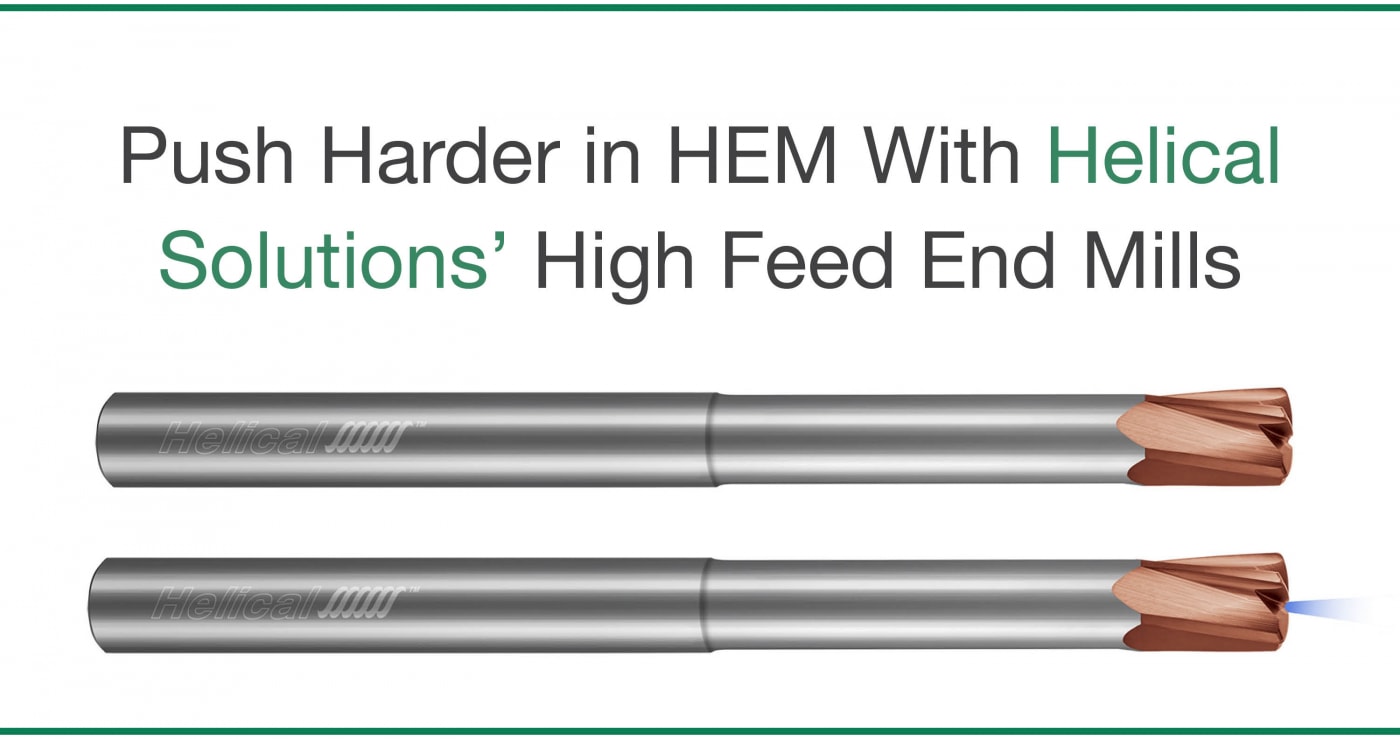The advertisement features two horizontal feed end mills, prominently displayed at the bottom of the image against a white background. Each mill showcases a brass or bronze-colored cutting surface on the right and a silver shank on the left, with the word "helical" printed on both shanks. Above the mills, black text reads: "Push Harder in H-E-M with Helical Solutions, High Feed End Mills," with "Helical Solutions" highlighted in green. At the top and bottom of the image, there are subtle green lines framing the ad. The design includes the Helical Solutions logo, characterized by six slashes with curved ends. The overall presentation suggests a professional and technical promotion of high feed end mills manufactured by Helical Solutions.